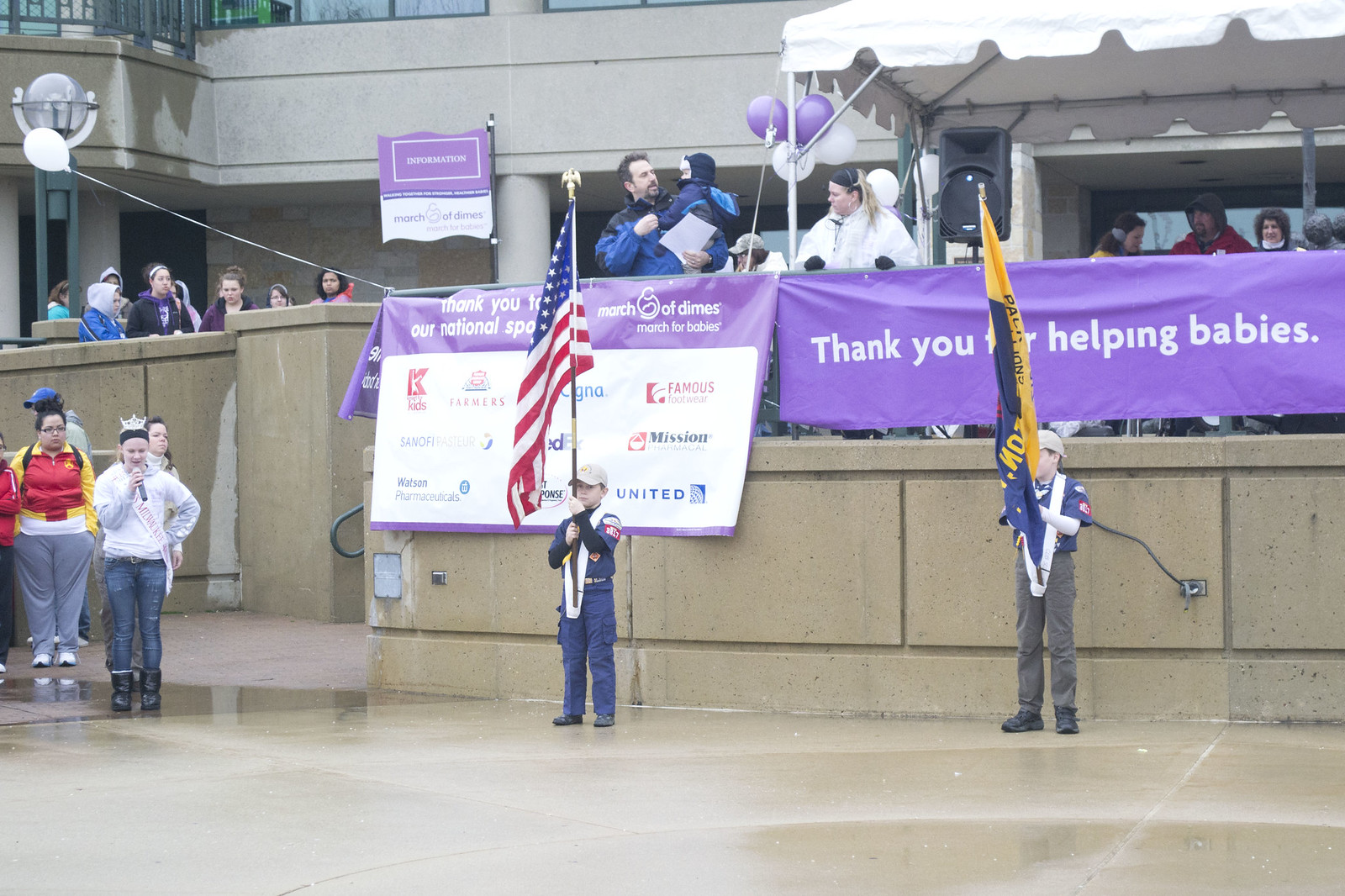In this outdoor photograph taken during the daytime, the scene unfolds after a recent rain, evidenced by the wet cement walls of the building in the background and the soaked ground. The setting hints at some form of ceremony or parade, possibly a March of Dimes event, marked by the prominent banners and sponsor logos. 

In the lower left corner, a girl of Caucasian descent, crowned and adorned with a sash reading "Miss Milwaukee," stands in a small puddle, her head bowed as she sings into a microphone. To her right, two Boy Scouts stand at attention, each holding a flag- one the American flag and the other likely the Milwaukee flag. Behind them, a young man cradling a baby stands next to a young woman, adding a touch of everyday life to the formal scene.

A white stage, elevated behind a border wall of damp cement, is decorated with purple and white balloons and banners. These banners carry messages such as "Thank you for helping babies," along with information about the March of Dimes and its sponsors, which include Farmers Insurance, Mission, United, Famous Footwear, Watson Pharmaceuticals, Cigna, and FedEx. The ceremony, organized in front of a building that might be a hospital, also features a significant amount of speaker equipment, indicating the importance and formality of the event.